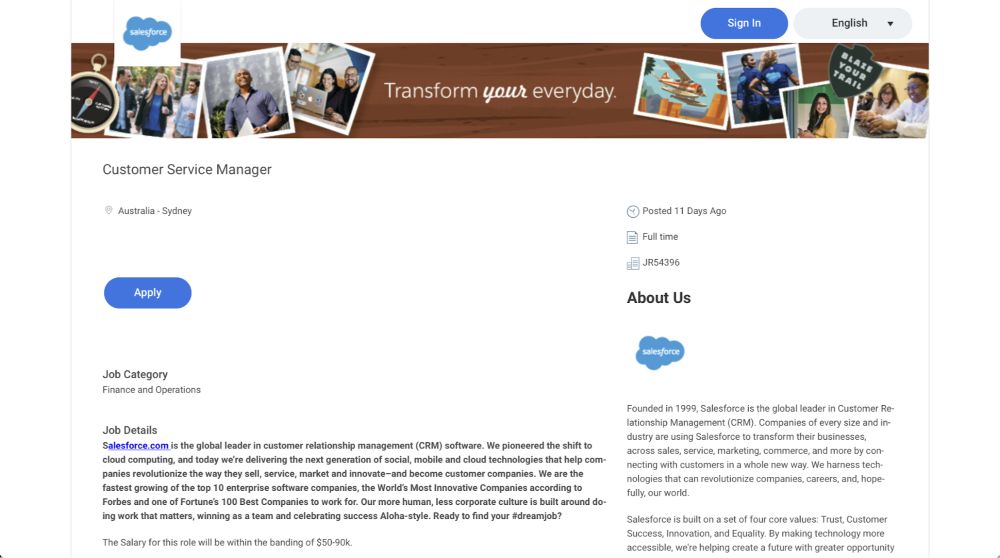This image showcases a job listing on a web page for the position of a Customer Service Manager located in Sydney, Australia. The top section prominently features the headline "Transform Your Everyday," inviting potential applicants to consider this opportunity. Below the headline, the job title "Customer Service Manager" is listed, followed by the location, "Australia, Sydney," and an "Apply" button. The job was posted 11 days ago and is categorized as a "Full Time" position with the reference code "GR54396."

The job falls under the categories of "Finance and Operations." Below this, details about the hiring company, Salesforce.com, are provided. The description highlights Salesforce.com's leadership in customer relationship management (CRM) software and its pioneering efforts in cloud computing. The company emphasizes its delivery of next-generation social, mobile, and cloud technologies, which are designed to help companies revolutionize their sales, service, marketing, and innovation processes, turning them into customer-centric companies.

Additionally, it notes that Salesforce.com is the fastest-growing company among the top 10 enterprise software firms, recognized as the world's most innovative company by Forbes and one of Fortune's 100 Best Companies to Work For. The company prides itself on fostering a "One more human, less corporate" culture focused on meaningful work.